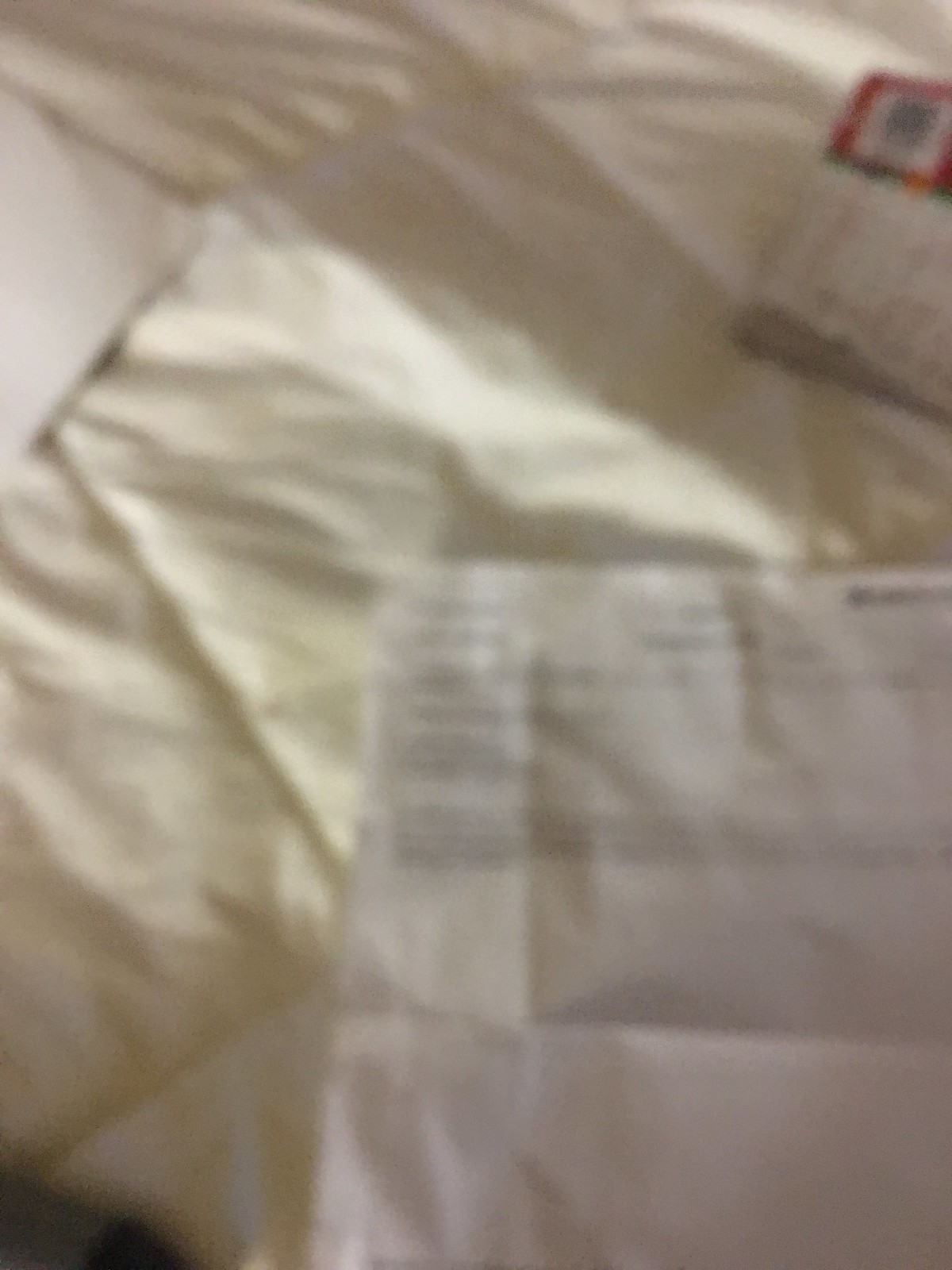A somewhat out-of-focus photograph captures a yellowish-white comforter or sheet draped over a bed. Scattered across the bedding are several papers and a book. In the bottom right-hand corner, a white sheet of paper with indistinguishable black text and markings can be seen, its details blurred. In the upper right-hand corner sits a book, featuring a white base with red and green sections towards the top, and what seems to be a UPC code, although the clarity is lacking to confirm. The overall image is slightly blurry, making the finer details difficult to distinguish.